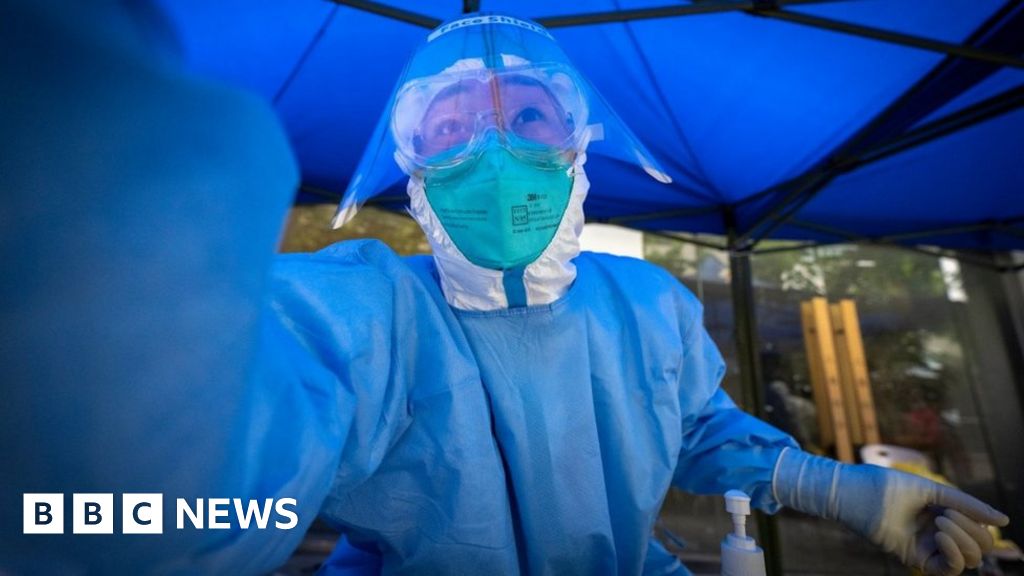A person, presumably a healthcare worker, is depicted wearing a full-body blue protective suit that resembles plastic material. They are equipped with gloves and their left hand is positioned to the left side of the image, while their right hand appears to be gripping a screen. The individual is protected by a clear face shield labeled "Face Shield" at the top, and beneath it, they wear large protective goggles over their regular glasses. Their attire also includes a light blue-green face mask, complemented by a white head covering that secures their hair. Additionally, a white apparatus, resembling a pump, is visible near their left hand. The background reveals a series of windows that could be part of a shop or facility. A tarp, likely blue, is suspended above the person. The bottom left corner of the image has the "BBC News" logo.